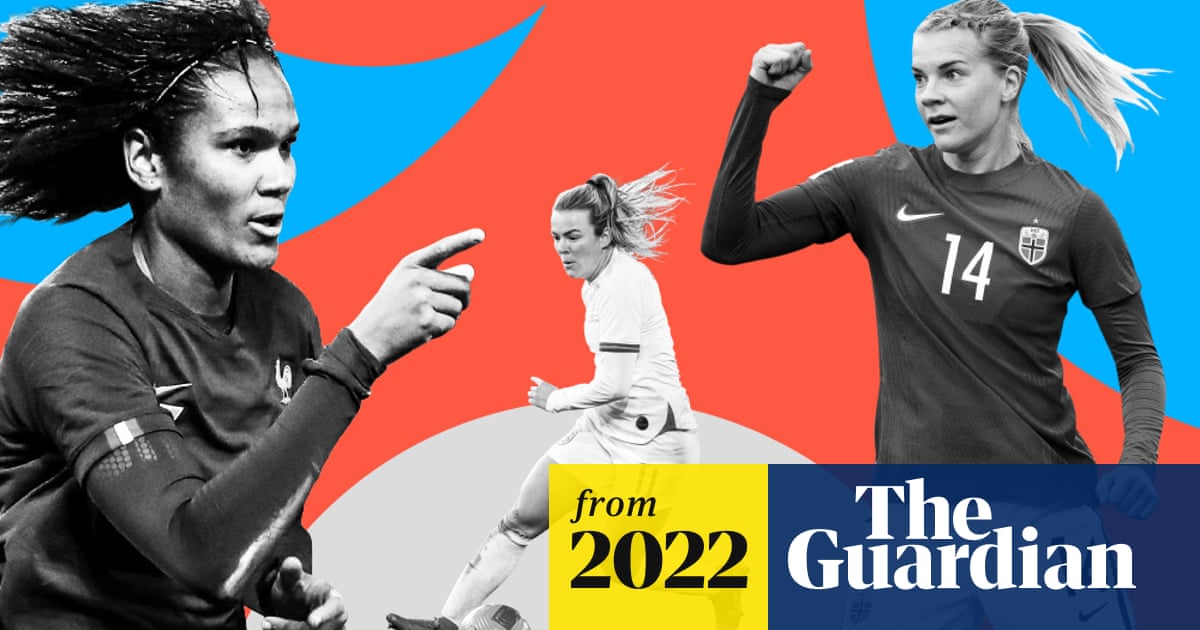This is an advertisement poster from The Guardian, dated 2022, which appears to promote women's soccer. The poster features three female athletes against a vibrant background of blue, red, and white geometric shapes. 

On the right, a blonde-haired woman, wearing a dark gray Nike jersey with the number 14 and a crest possibly from Sweden, Denmark, or Norway, is shown pumping her fist with determination. Her hair is tied back in a ponytail.

The center athlete, dressed in a white soccer jersey and shorts, has her hair tied in a ponytail and exudes intensity as she appears to be running, as if chasing a ball.

On the left, a Black woman with shoulder-length hair flowing behind her is depicted running and pointing forward. She is clad in a dark-colored top, suggesting active participation in the game. 

The design also incorporates The Guardian's logo in a blue section at the bottom right, adjacent to a yellow rectangle that confirms the 2022 publication date.